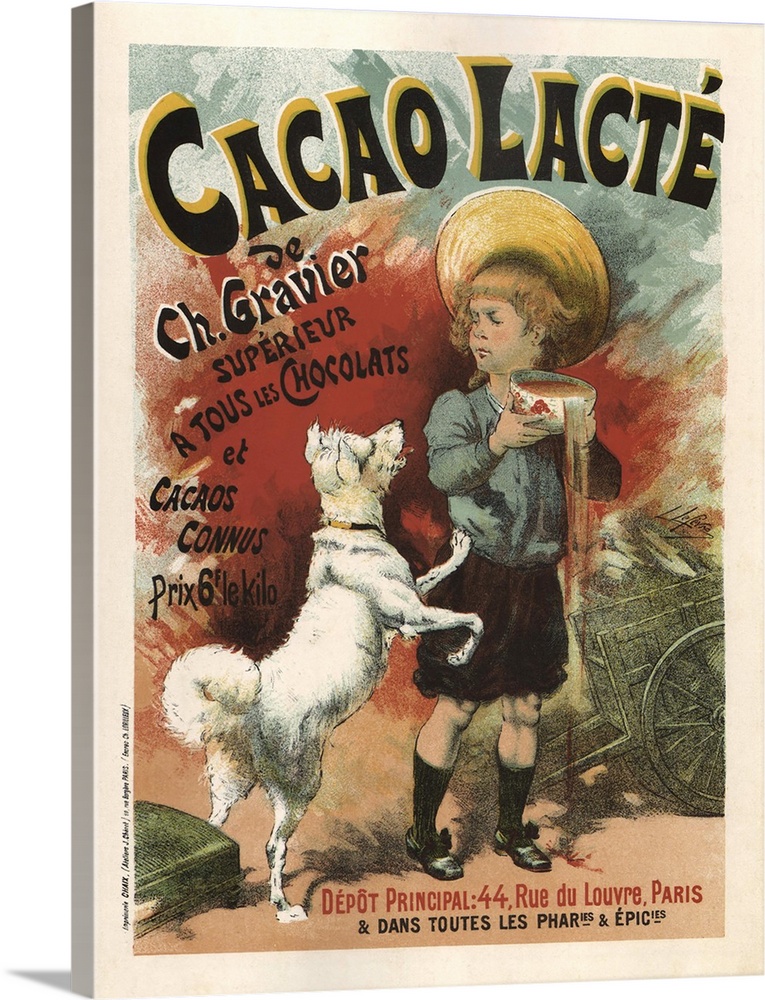The image appears to be a vintage-style advertisement or poster, crafted to look like it's stretched around a canvas on a white background with a drop shadow to the bottom left. At the top of the image, in large, bold, black letters, it reads "Cacao Lactée." Below this title, on the left side of the canvas, there are additional French text details which appear to continue downwards. 

Central to the artwork is a painting of a small child with orange, wavy hair, wearing a wide-brimmed brown hat, a teal-colored shirt, black shorts or bloomers, knee-high black socks, and black shoes with bows. The child is holding a large white bowl with a red design, possibly filled with chocolate, that is spilling over the right side. To the left of the child, a small white dog is standing on its hind legs with its front paws resting on the child's hip, eagerly looking up at the bowl with its mouth open, as if begging for a taste. The child is tilting the bowl away, seemingly to keep it out of the dog's reach. 

In the background, to the right, an old-fashioned wooden wheelbarrow or wagon is partially visible, adding a quaint, rustic element to the composition. The image is bordered by a light frame that enhances its vintage appeal.